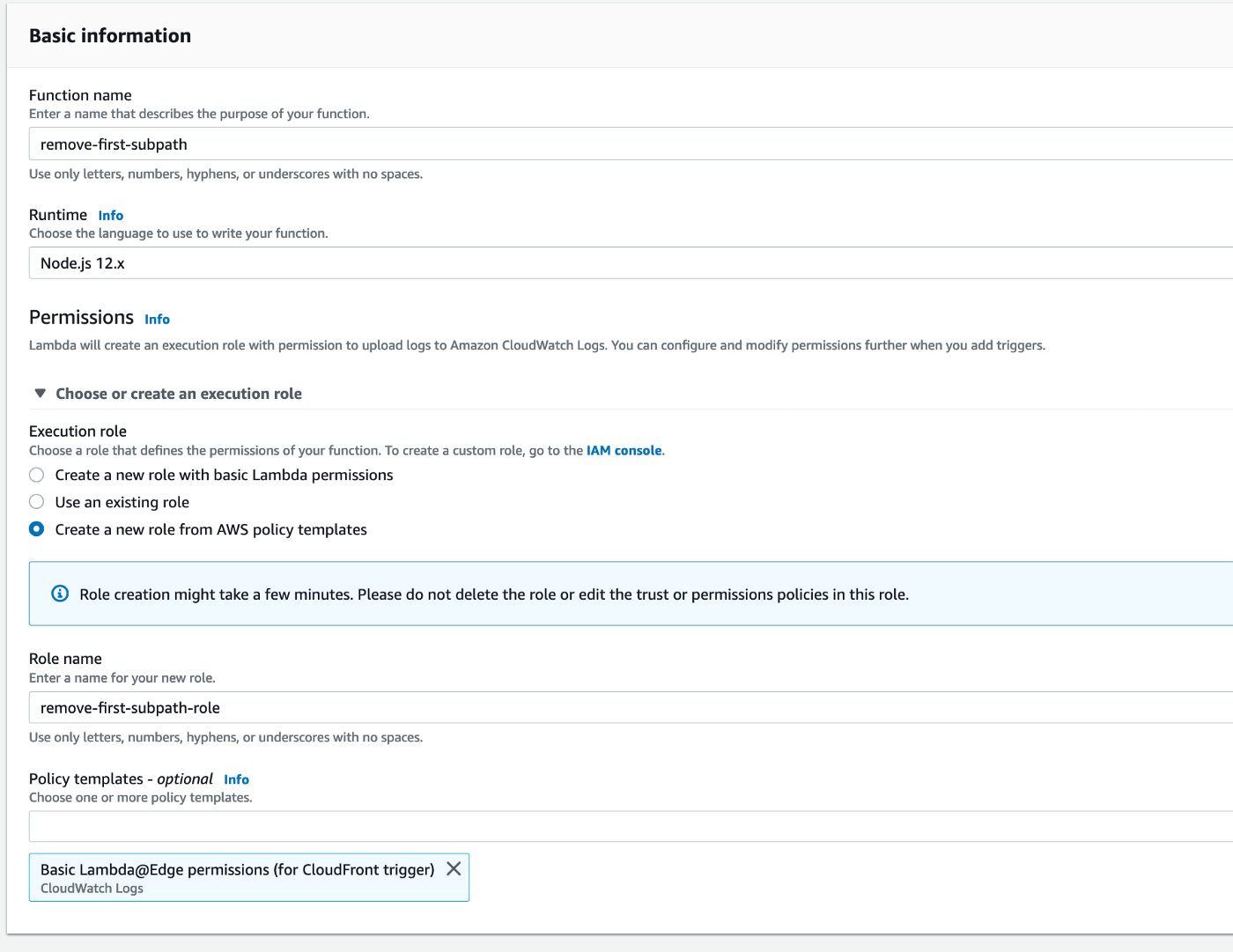The image depicts a detailed configuration screen for creating a Lambda function within a cloud platform interface.

In the upper-left corner, there's a section titled "Basic Information." Beneath this heading is a label, "Function Name," followed by an instructional text in smaller font: "Enter a name that describes the purpose of your function." To the right is a long input field containing the text "remove-first-subpath."

Further down, there's a section labeled "Runtime" with a blue "Info" link adjacent to it. Below this, it reads, "Choose the language to use to write your function," accompanied by another rectangular input field that contains "node.js12.x."

Next is a section labeled "Permissions," again with a blue "Info" link next to it. Beneath this, it instructs the user to "Choose or create an execution role." Following this instruction is a large, light blue rectangle with a cautionary note: "Role creation might take a few minutes. Please do not delete the role or edit the trust or permissions policies in this role."

Continuing down, the screen prompts with "Role Name." There's an input field below this containing "remove-first-subpath-role."

Finally, at the bottom of the screen, inside a blue rectangle, is the text "Basic Lambda@Edge.Permissions (for CloudFrontTrigger)."